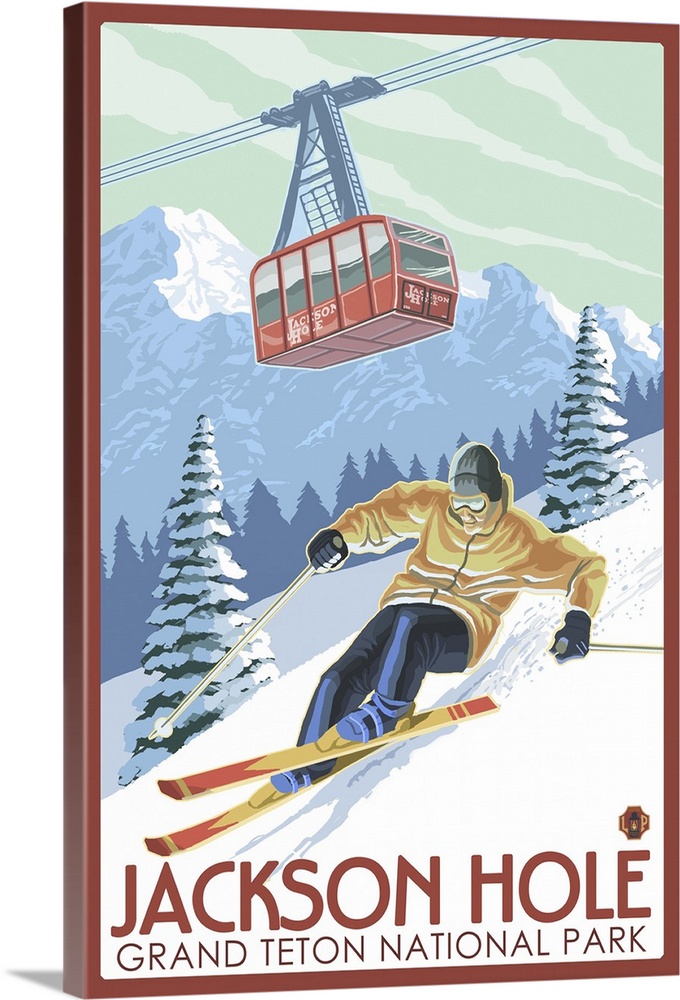The image appears to be a visually striking poster or advertisement depicting a dynamic skiing scene at Jackson Hole in Grand Teton National Park. A male skier, dressed in a vibrant yellow jacket, dark blue pants, yellow and red skis, and equipped with ski poles, is the central figure, careening down a snow-covered mountainside. Above him, a red gondola with side windows, seemingly able to carry multiple passengers, traverses the sky. Majestic, snow-draped mountain peaks rise in the distance, contrasting the skier's slope, which is dotted with snow-laden evergreen trees. The bold red text at the bottom of the image reads "Jackson Hole," with "Grand Teton National Park" positioned just below it, anchoring the scene. The entire poster has a slightly three-dimensional, framed appearance with a shadow effect on the white background, suggesting it might be a digitally rendered artwork.